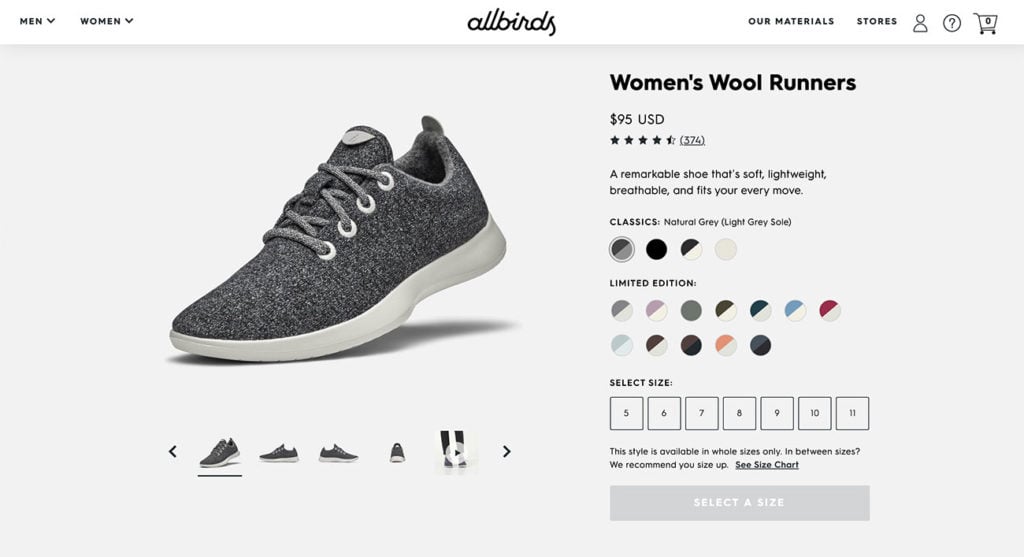The webpage displayed is from an online store listing various bird-themed shoes, with two primary navigation tabs at the top for "Men" and "Women." On the right side of the page, sections for "Our Materials" and "Stores" can be found. The current selection is on women's Wool Runners, priced at $95. These shoes have garnered an impressive rating of 4.5 stars from 374 reviews. Described as a remarkable shoe, it boasts features such as softness, lightweight construction, breathability, and a design that fits every move. The primary color available is Natural Gray with a Light Gray sole, but it also comes in Black, Black and White, and pure White. Limited edition colors are also available, including Blue and White, Red and White, Pink and White, Light Mint Green, and Orange and White.

The sizes range from 5 to 11, available only in whole sizes. For those between sizes, it is recommended to size up. There is an option to view a size chart by clicking a small arrow, which also allows viewing the shoe from various angles. At the bottom of the page, customers can select their desired size from the available options.